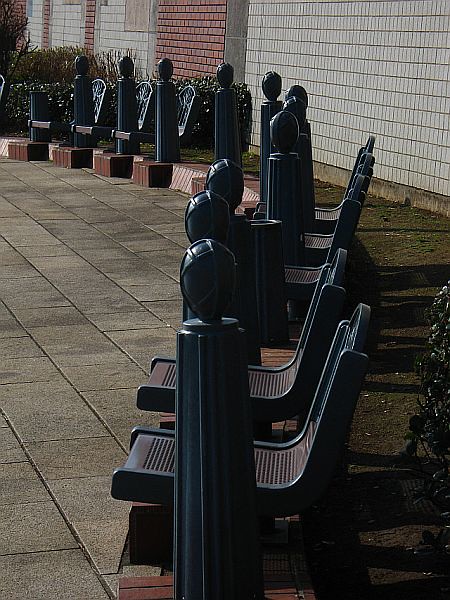The image depicts an outdoor seating arrangement with approximately ten individual dark blue resin chairs, each adorned with a back design that hints at a tree pattern and holes in the seats. These chairs are interspersed with black metal posts, similar to public safety bollards often seen at store fronts. The seating area, bordered by square concrete slabs, resembles a bus stop or a public waiting area. The chairs form a long line, with occasional gaps between them, situated along the edge of a patio or sidewalk. Behind the chairs, there's a strip of grass accompanied by bushes, leading back to a backdrop that alternates between red brick and white tile sections, giving the scene a structured and urban feel. The overall impression is reminiscent of seating outside a sports stadium or an auditorium.